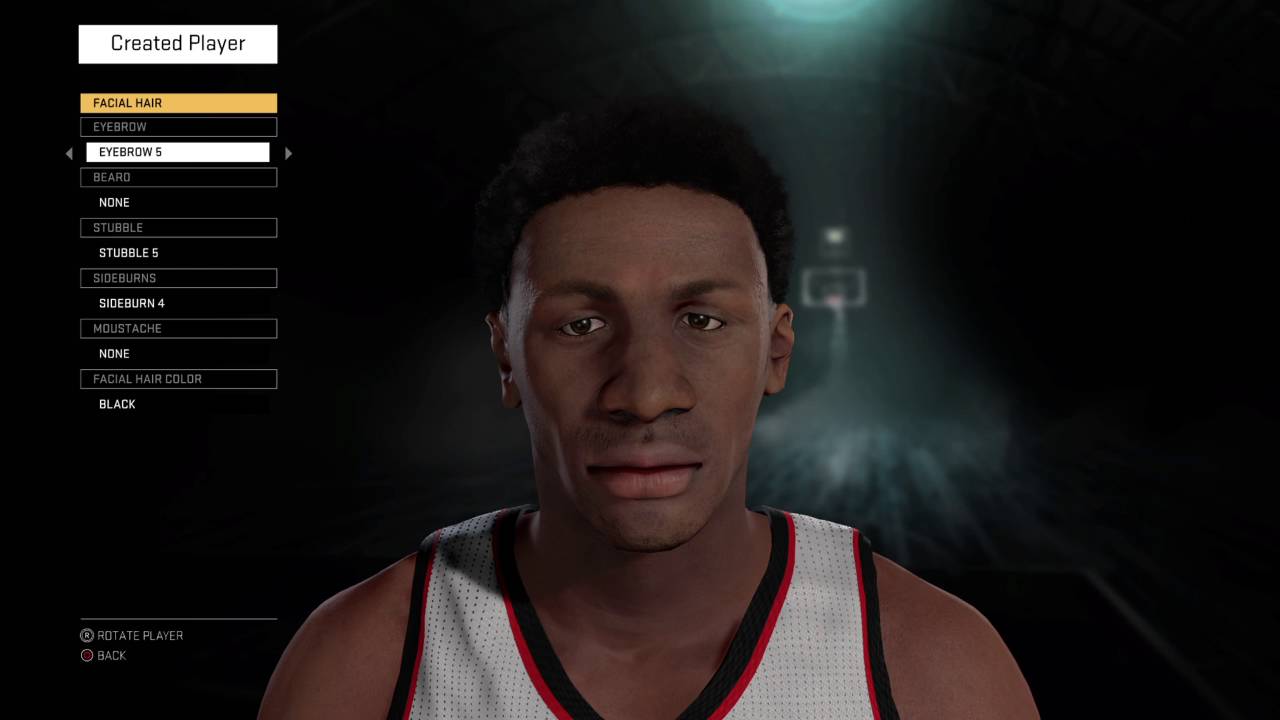The screenshot from the video game features a created character, a Black man with a small afro haircut, looking directly at the camera. He is wearing a white tank top accented with black and red stripes around the armholes and collar. Behind him, a light on the ceiling illuminates the scene, casting shadows through the rising smoke. Additionally, a basketball hoop is visible, adding a sporty theme.

Various customization options are displayed on the left side of the screen in distinct colored boxes. A white box titled "Created Player" leads the list, followed by a yellow box labeled "Facial Hair." Proceeding downward, a series of black and white boxes offer further customization features: "Eyebrow," with the specific selection "Eyebrow 5"; "Beard," which currently shows "None"; "Stubble," set to "Stubble"; "Sideburns," set to "Sideburns"; "Mustache," marked as "None"; and "Facial Hair Color," specified as "Black."